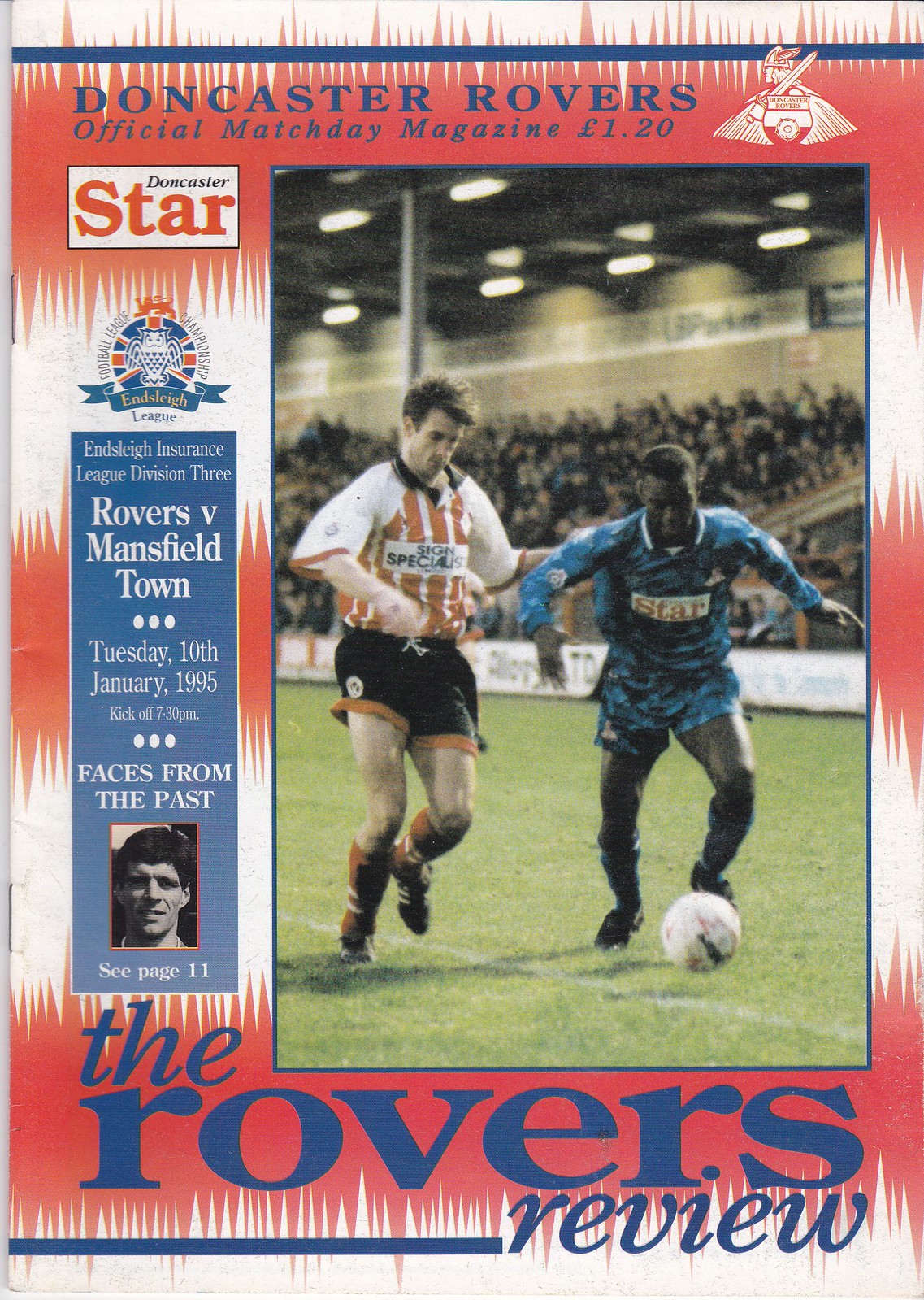The image is a vintage poster for a football match, presented as the cover of the official Match Day magazine of the Doncaster Rovers, titled "The Rovers Review." Retailing for £1.20, the magazine cover, which features a jagged red and white background with blue accents and medium-toned blue font, highlights an upcoming game against Mansfield Town scheduled for Tuesday, January 10th, 1995, with a kickoff at 7:30 p.m.

Prominently displayed on the right side of the cover is a black-and-white photograph of two players in action, one white gentleman wearing a white jersey with red stripes, black shorts with red accents, red socks, and black cleats, and a black gentleman in a blue long-sleeve jersey with the word "Star" on it, blue socks, and black cleats. This image captures the competitive spirit of the match.

On the left side of the cover, a white box at the top reads "Doncaster Star," followed by the Ensley League emblem, which incorporates the UK flag and a graphical depiction of an owl. Below, in a blue box with white text, the highlighted match details are reiterated as "Ensley Insurance League Division 3, Rovers vs. Mansfield Town, Tuesday, January 10th, 1995, 7:30 p.m." Additionally, a section labeled "Faces from the Past" under this box introduces a featured article about a past player, directing readers to page 11 for more details. The overall design, indicative of its 1995 origin, carries a nostalgic vintage aesthetic.